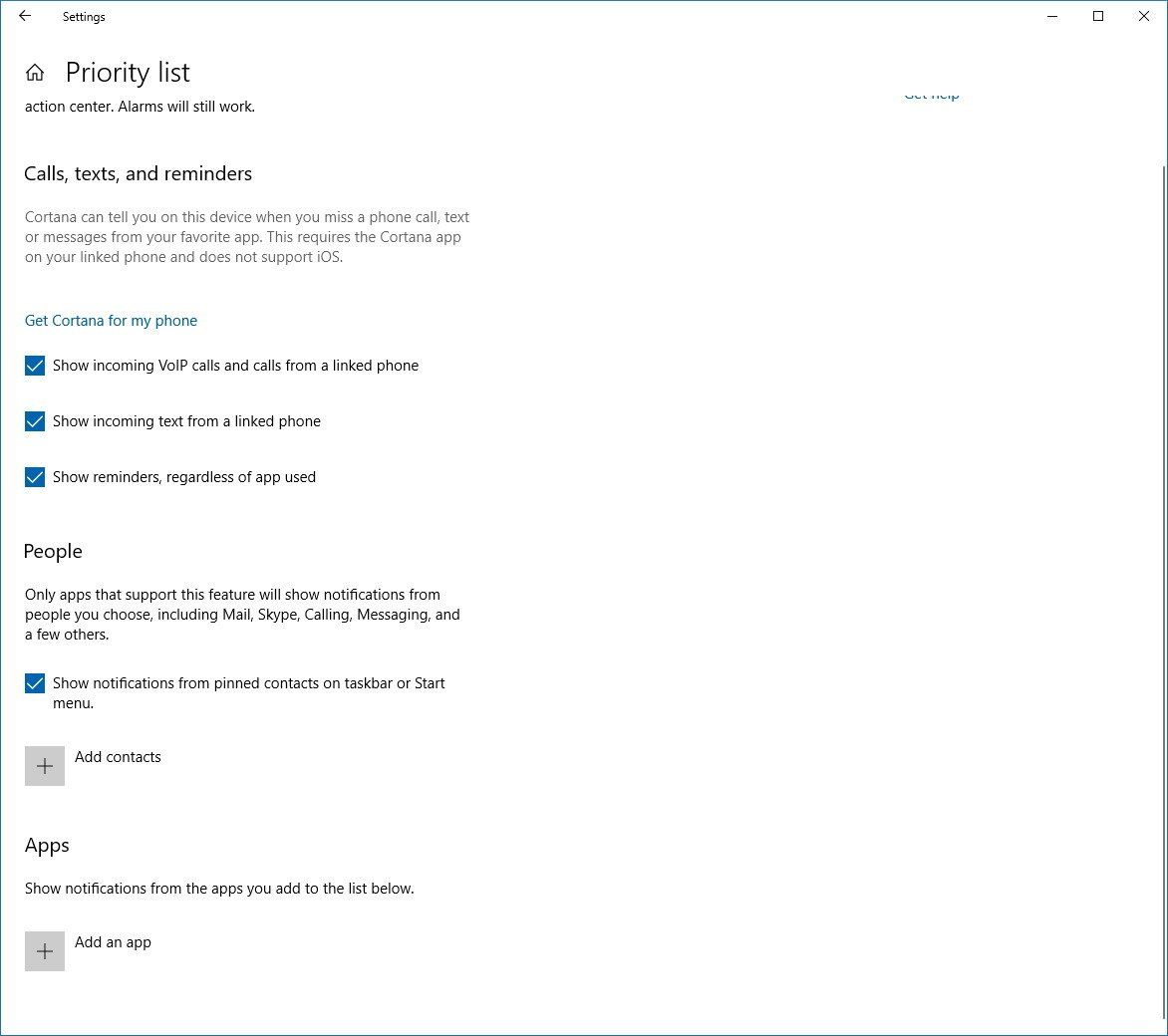**Detailed Caption:**

The image displays a screenshot of a "Priority List" under the "Settings" menu. The top section features an icon of a house next to the heading "Priority List." Below this, the "Action Center" is mentioned, noting that alarms will continue to function. The next section, titled "Calls, Texts, and Reminders," highlights how Cortana can notify the user on this device about missed calls, texts, or messages from preferred apps. This feature necessitates having the Cortana app on a linked phone and isn't compatible with iOS devices. There is a clickable link labeled "Get Cortana for my phone."

Further down, three blue boxes with white check marks underscore options for notifications. The options read: "Show incoming VoIP calls and calls from a linked phone," "Show incoming texts from a linked phone," and "Show reminders regardless of app used."

The "People" section follows, explaining that only apps supporting this feature will display notifications from chosen contacts, including apps like Mail, Skype, Calling, Messaging, and a selection of others. An option allows users to "Show notifications from pinned contacts on the taskbar or start menu." A plus sign then invites users to "Add contacts."

At the very bottom, there is an option to "Add an app."